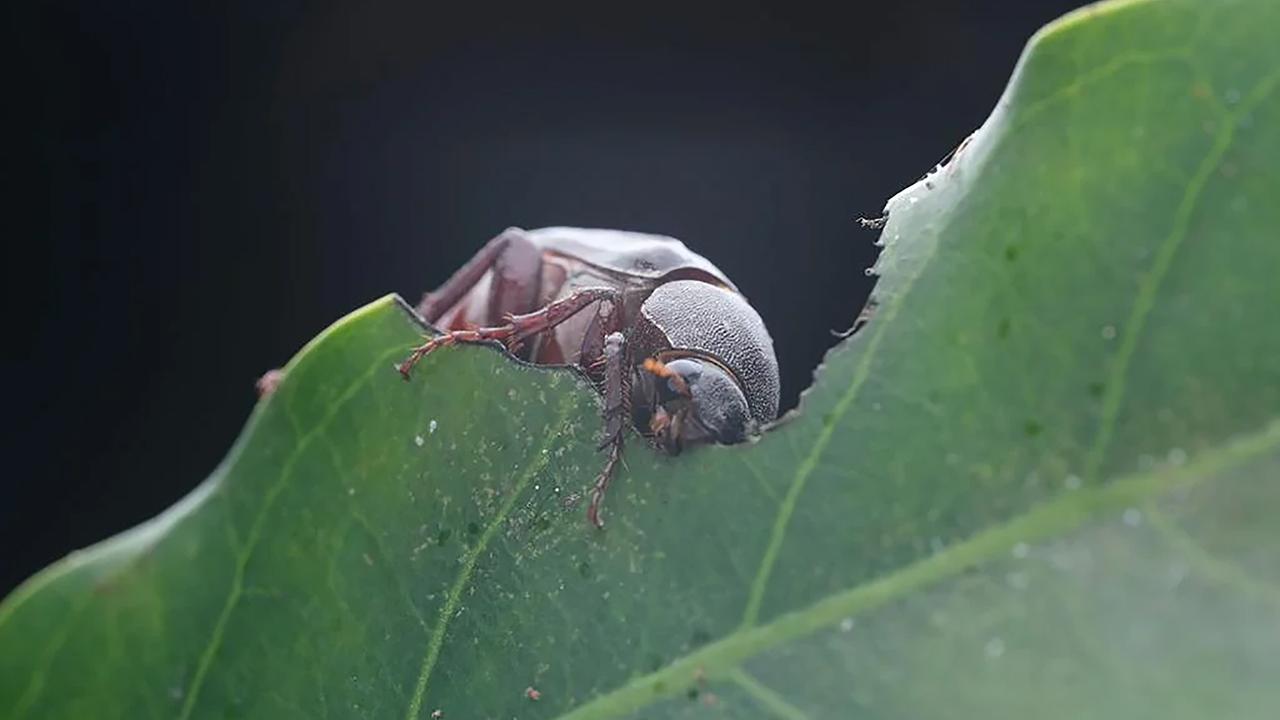The image is a detailed, close-up photograph taken outdoors, featuring an insect on a green leaf. The insect, possibly a beetle, displays a black head and a segmented, sturdy back shell, with its abdomen extending behind it. The beetle is characterized by its black and brown coloration with a hint of orangish tinge near its head. We can clearly observe two of its long, hairy legs with segmented portions situating the insect on the leaf. The photograph highlights the beetle actively eating the leaf, creating a distinctive U-shaped bite mark. The green leaf features a prominent center vein with two side veins and a reticulate pattern that provides a textured backdrop to the beetle's activity. This intricately veined leaf diagonally spans from the lower left to the upper right corner of the image. The background of the photograph is completely black, ensuring all attention is drawn to the feeding beetle and the detailed structure of the leaf.